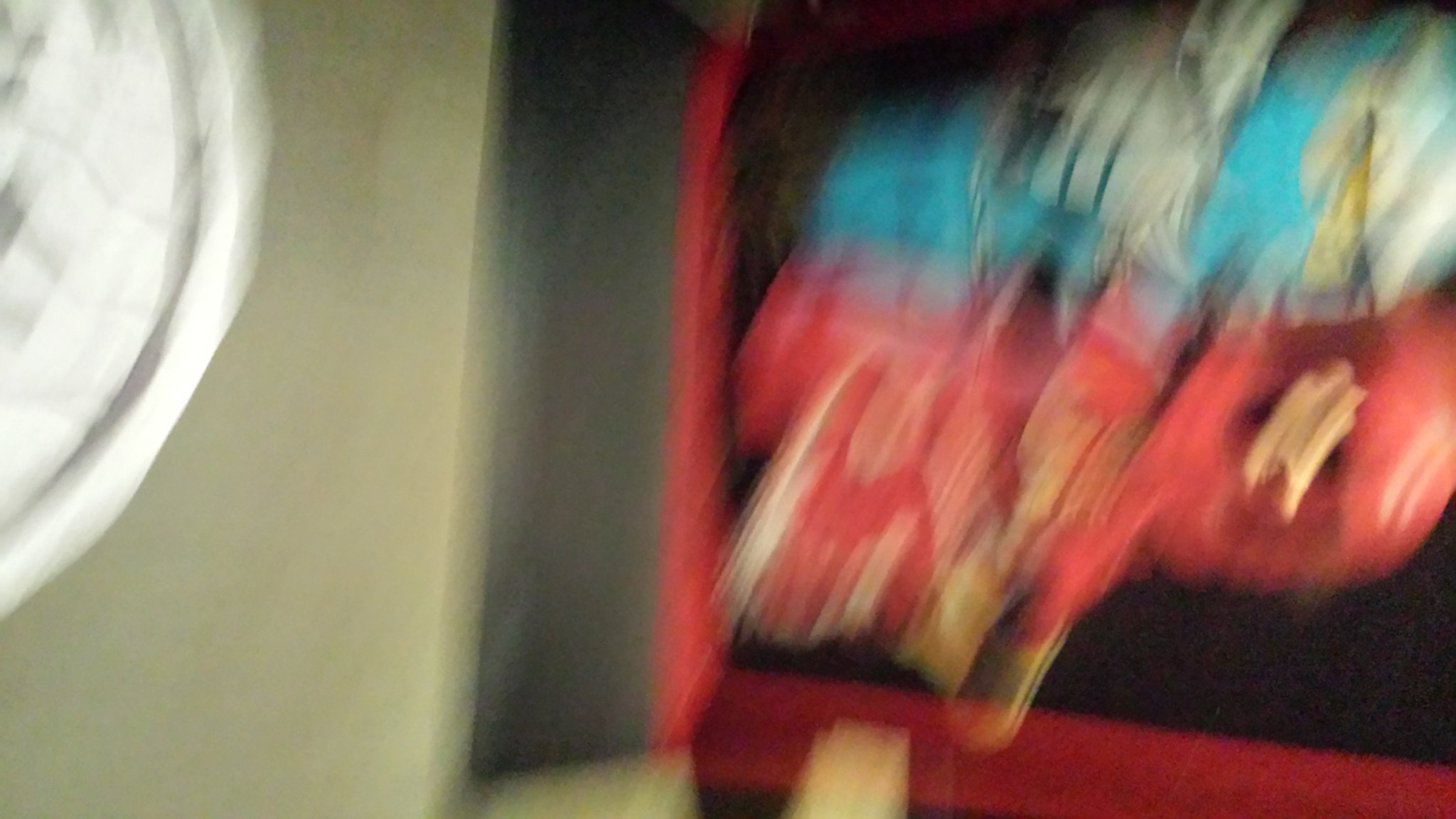The photograph is heavily blurred, making it difficult to discern specific details. On the left side of the image, there appears to be a vertical line, possibly signifying a light fixture, partially visible with a hint of a white circle adorned with dark lines. To the right, there is an object that resembles a red basket or shelf holding what seem to be bag-shaped items. The bottom bag displays a red and white color scheme with a beige section, while the bag above features a light blue hue with wide white and black stripes, also accented by a beige segment.